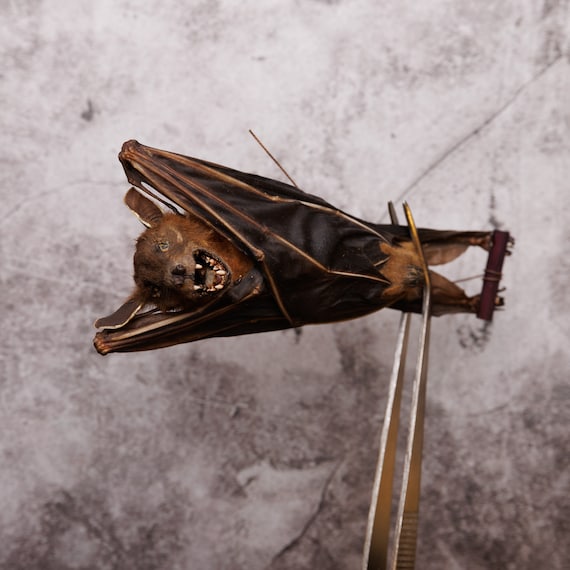The image depicts a mummified bat, brownish-black in color, oriented horizontally with its head to the left and its feet to the right. The bat's mouth is open, displaying four distinct fangs—two on the top and two on the bottom. Its wings are tightly wrapped around its body, emphasizing the small pointed ears and a furry head. Silver tweezers hold the bat aloft by its feet, which are attached to a small brown stick. The bat is set against a gray and white dirty wall, and the absence of any text highlights the eerie, detailed nature of the bat's preserved state. The subtle contrasts of off-white, gray, black, brown, dark brown, and silver accentuate the bat's striking, mummified features, creating a hauntingly realistic impression.